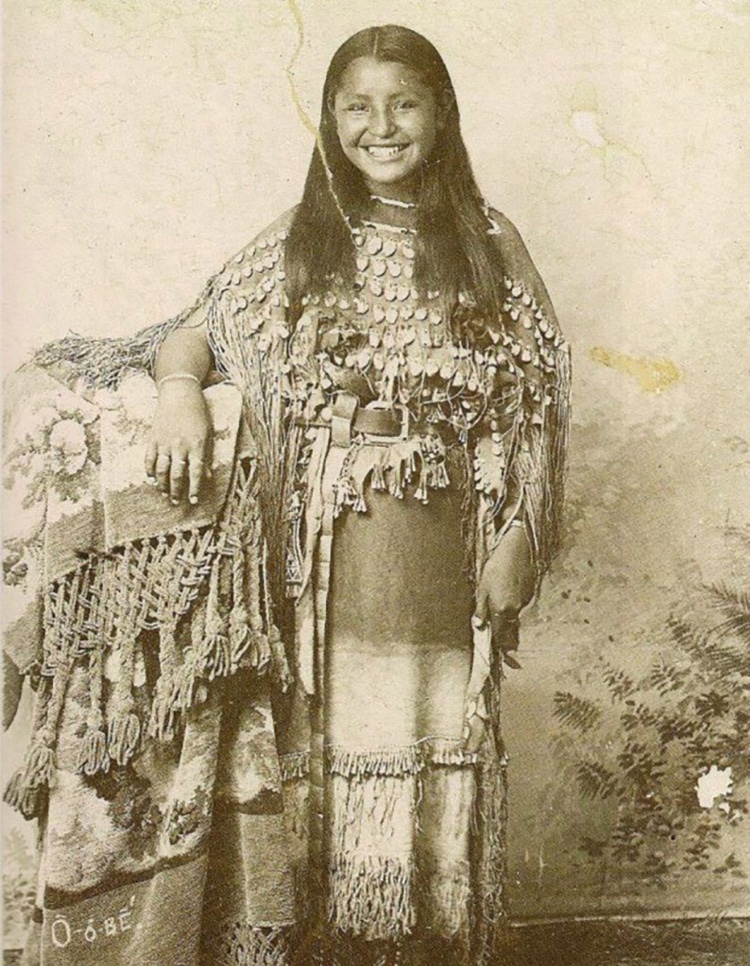The image is a sepia-toned, aged photograph of a young Native American girl, likely in her early teens. Her long, dark hair cascades down as she stands with a cheerful smile, her left elbow resting on a bench or stool draped with a frilly, patterned blanket. She is dressed in traditional attire adorned with fringe and what appear to be beads or medallions across the top, cinched at the waist with a belt. The dress features a tiered color transition from cream to brown and back to cream at the bottom. The photograph itself has visible creases and tears, especially near the top center, adding to its antique appearance. The background is plain with worn-out wallpaper, further emphasizing the picture's aged and rustic charm.